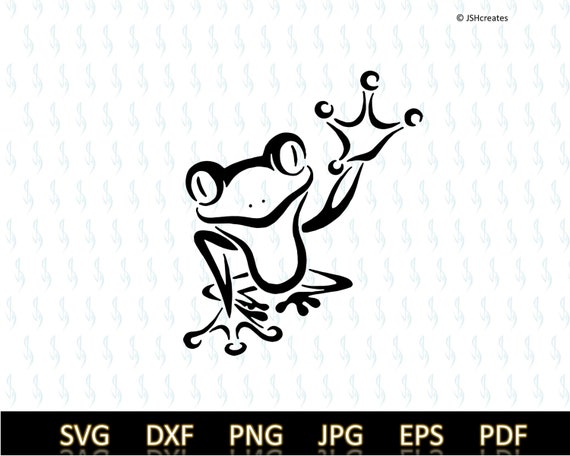The image depicts a detailed graphic art of a frog, likely a stock design or emblem. In the upper right corner, the text "JSH creates" along with a copyright mark is prominently displayed. The background is filled with repeating blue, squiggly lines or logos, creating a textured backdrop. 

The central figure is a striking black frog with exaggerated features, including bulgy eyes with slits, two noticeable nose holes, and a wide mouth. The frog is positioned with one arm raised, showcasing its three fingers and a thumb, while its other foot and two back legs remain grounded. 

At the bottom of the image, a black rectangular bar stretches across, with the file formats SVG, DXF, PNG, JPG, EPS, and PDF written in white or light yellow text. This suggests the image is available in multiple digital formats. The overall design is intricate and eye-catching, emphasizing the outlined and artistic representation of the frog.